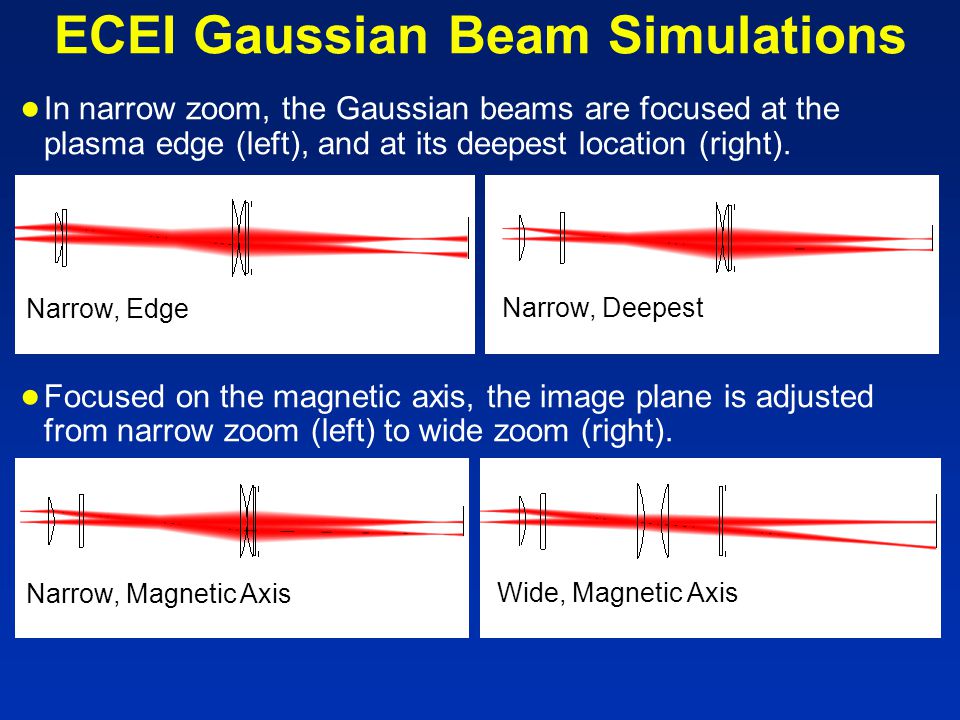This detailed image poster, titled "ECEI Gaussian Beam Simulations," features a dark blue square-shaped background with prominent yellow heading text at the top. The heading reads "ECEI Gaussian Beam Simulations." Beneath the heading are two yellow bullet points, both centered on the page and in white font.

The first bullet point explains, "In narrow zoom, the Gaussian beams are focused at the plasma edge (left) and at its deepest location (right)." Directly below this text are two side-by-side white rectangular graphics. The left graphic is labeled "narrow edge" and the right one is labeled "narrow deepest." Both graphics show red Gaussian beam simulations traversing from the left to the right sides of the rectangles.

The second bullet point states, "Focused on the magnetic axis, the image plane is adjusted from narrow zoom (left) to wide zoom (right)." Below this text are two additional side-by-side white rectangular graphics. The left graphic is labeled "narrow magnetic axis" while the right one is labeled "wide magnetic axis," each depicting red beams extending from the left to the right of the rectangles.

Structurally, the layout of red beam simulations is organized in four distinct white rectangular blocks, with two blocks in the first row and two in the second row, creating a clear and systematic representation of the Gaussian beam simulations.